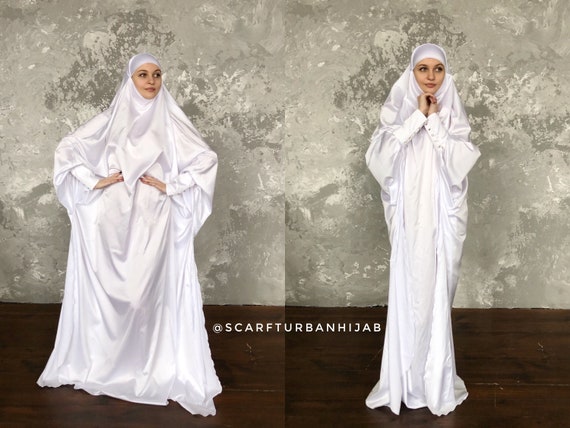The image is a horizontal format featuring two side-by-side photos of a young woman with a slight model build, dressed in a long, white, silk hijab that covers her entire body except for her face and hands. The gown, or hijab, is long-sleeved with cuffs and buttons. In both images, she has a concerned expression and is looking to the right. On the left, she stands confidently with one hand on her hip, showcasing the flowing nature of her garment. On the right, she adopts a more conservative pose, with her hands together and placed under her chin. The background of both images features a greenish sponge painting effect, blending seamlessly across both photos, with a smooth, dark wood floor beneath her.